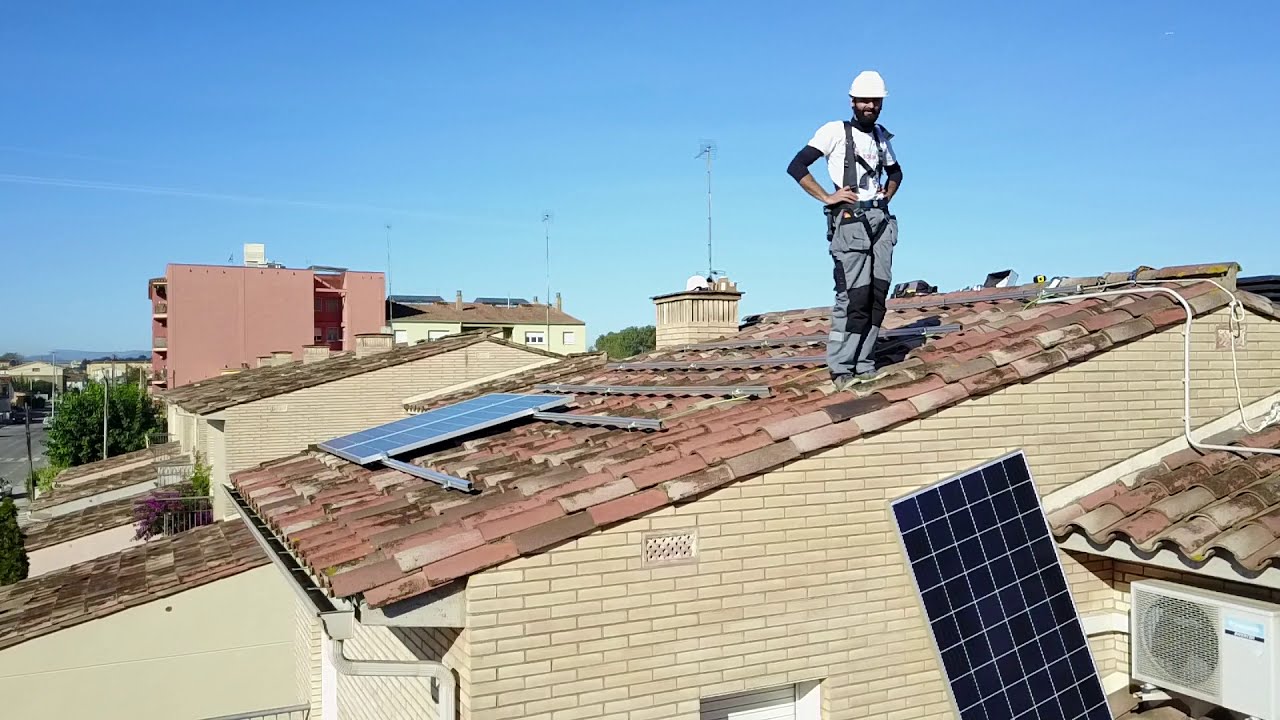A black man with a thick beard and a white hardhat stands confidently on a slanted rooftop, hands on his hips, smiling and looking content. He wears a white shirt, a black safety harness, and black sleeves that extend just below his elbows, paired with rave pants featuring black knee patches. The tiled roof under his feet ranges in color from orange to light brown, with some tiles appearing wet. Mounted solar panels are positioned behind him, and another solar panel leans against the light brown wall of the building, which features darker brown grout. An air conditioner unit is visible in the bottom right corner. In the distance, a cityscape with several rooftops and buildings unfolds, including a prominent orange building with a white square on top and various antennas. The sky above is a light blue with a visible contrail on the left side. The man appears to be a solar panel engineer or worker engaged in installing the panels, exuding a relaxed and content demeanor as he poses for the camera.